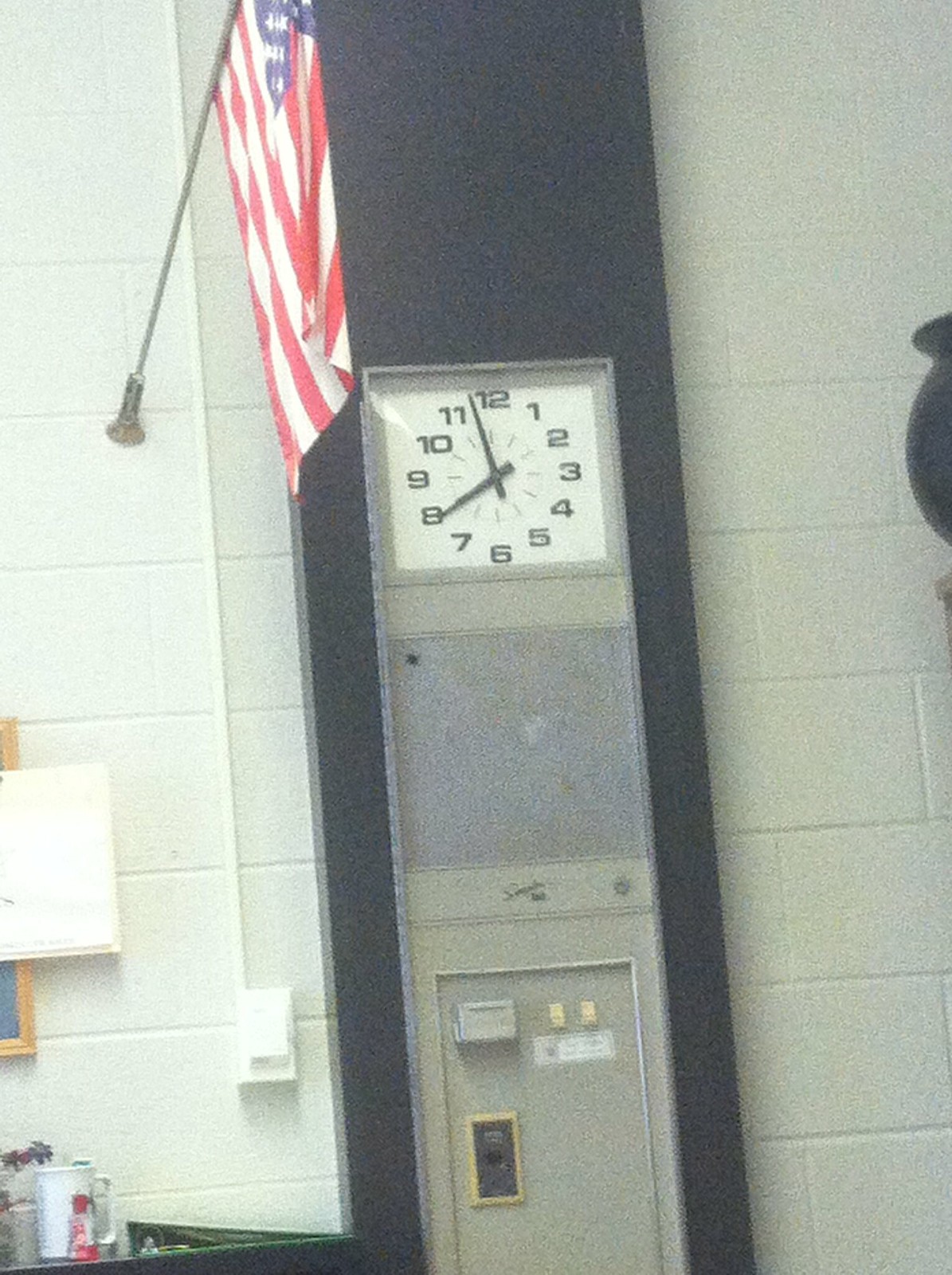The image depicts a robust, rectangular metal machine prominently mounted on a large, black-painted section of the wall, which appears to be made of wood. The machine features a large square clock at the top, providing a clear and functional display of time. Below the clock, in the center of the device, lies a substantial square speaker with a grey face at its bottom. Located towards the right, two distinct buttons are visible, suggesting operational functionality. On the top left side, there is a slot that seems designed for card insertion. Further down on the left side, there is a key mechanism housed within a black rectangle, accentuated by a yellow border, which indicates its importance and possible security function. The entire setup is mounted on a white-painted concrete wall, with the texture of the concrete bricks visibly detailed. To the left of the machine, a flag is hanging, adding a touch of decor and possibly indicating the location or significance of the room. The left side thickness of the machine can be discerned from the partial view provided, emphasizing its sturdy and solid construction.